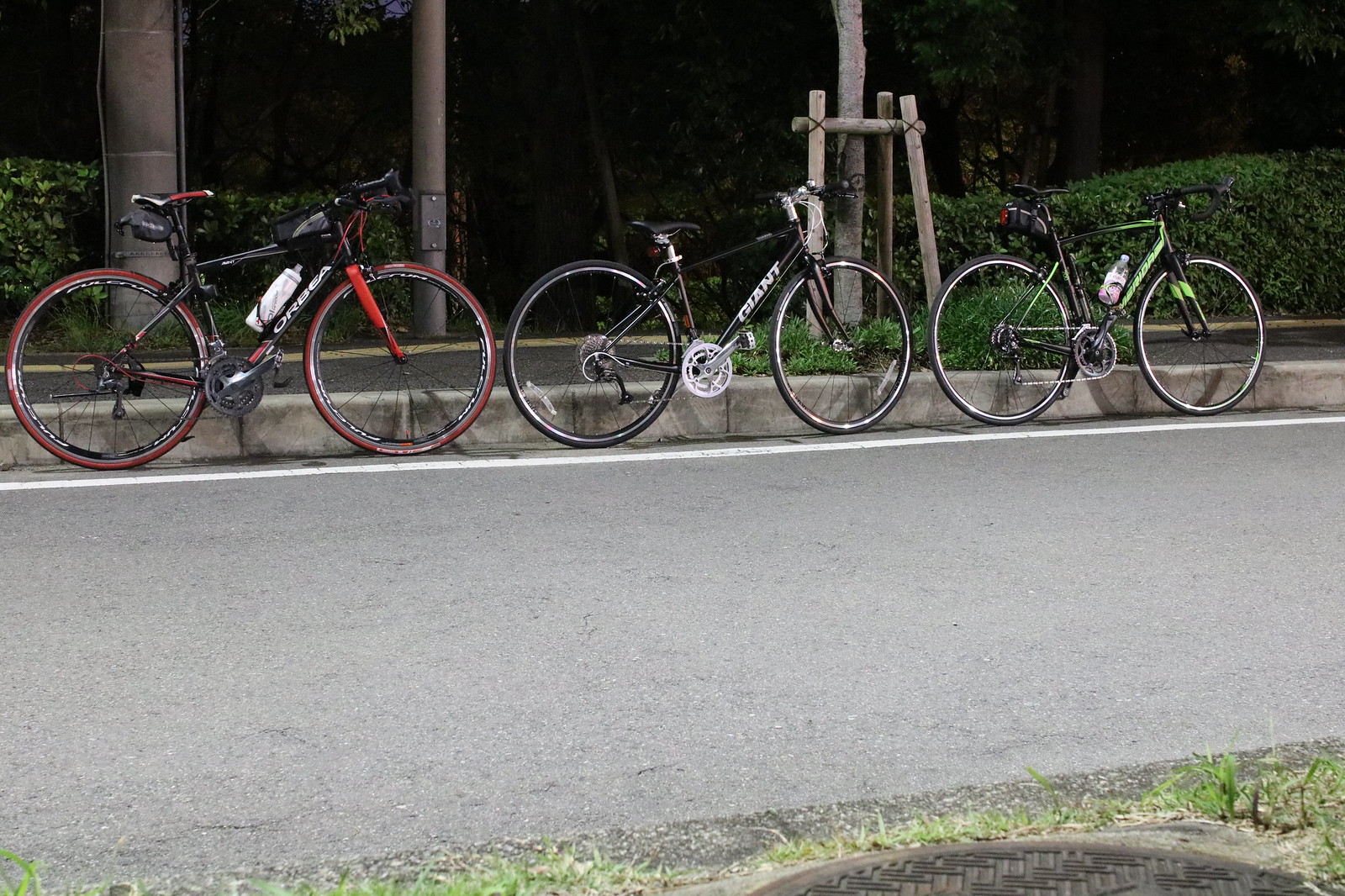This outdoor daytime photograph captures a row of three parked bicycles beside a light gray asphalt road. The road features a white stripe near the bikes, which are lined up end-to-end. In the lower right corner of the image, part of a sewer grate is visible. The first bicycle, on the left, is predominantly black with red accents, including a red frame, front spoke, seat highlights, and some red on the wheels. It bears the brand name "ORBEA" in white lettering and has a white water bottle attached. The middle bike is black with the brand name "GIANT" displayed in white text. The third bicycle, on the right, is black with green accents. All three bicycles have water bottles clamped to their frames. Behind the bikes, there's a mix of greenery, including bushes and the brown trunks of trees, and three utility poles clustered toward the upper left part of the photo. The background vegetation and well-lit conditions suggest the image was taken on a sunny day.